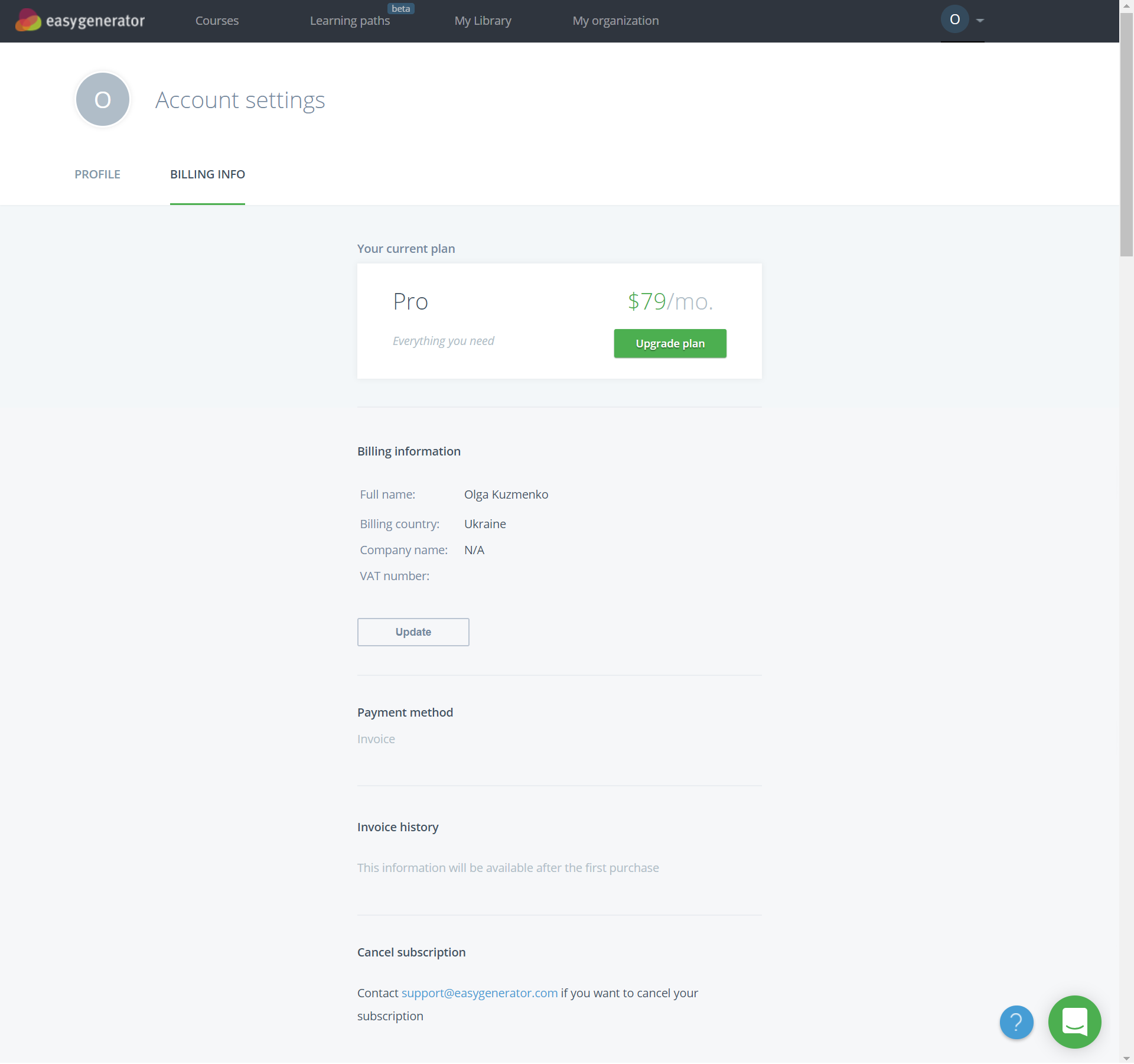The page features a user interface layout from EasyGenerator, complete with a black header at the top. On the left side of the header, "EasyGenerator" is displayed as one word, accompanied by a distinctive logo of multicolored circles. Sequentially to the right, the navigation menu includes options labeled: "Courses," "Learning Paths" with a "Beta" tag, "My Library," and "My Organization." On the far right of the header, there is a circle icon resembling an arrow.

Beneath the header, the main content area is set against a white background. Prominently, "Account Settings" is visible, accompanied by a blue-gray circular icon with a white interior. Below it are the subheadings "Profile" and "Billing Info," with "Billing Info" underlined in green.

The central section of the page, set against a light grayish-blue backdrop, begins with "Your Current Plan." Inside a white rectangle, it details the plan as "Pro, Everything You Need, $79/MO." A green button labeled "Upgrade Plan" follows this information. 

Further down, under "Billing Information," the user's details are specified: 
- Full Name: Olga Kuzmenko
- Billing Country: Ukraine
- Company Name: N/A
- VAT Number: None

An "Update" button is positioned below these details.

The "Payment Method" section mentions "Invoice" and "Invoice History," with a note that this information will be available after the first purchase. The section also includes a "Cancel Subscription" option with instructions to contact support at easygenerator.com for cancellation requests.

In the bottom right corner, two icons are present: a blue circle with a white question mark for help and a green circle featuring a chat bubble for customer support.